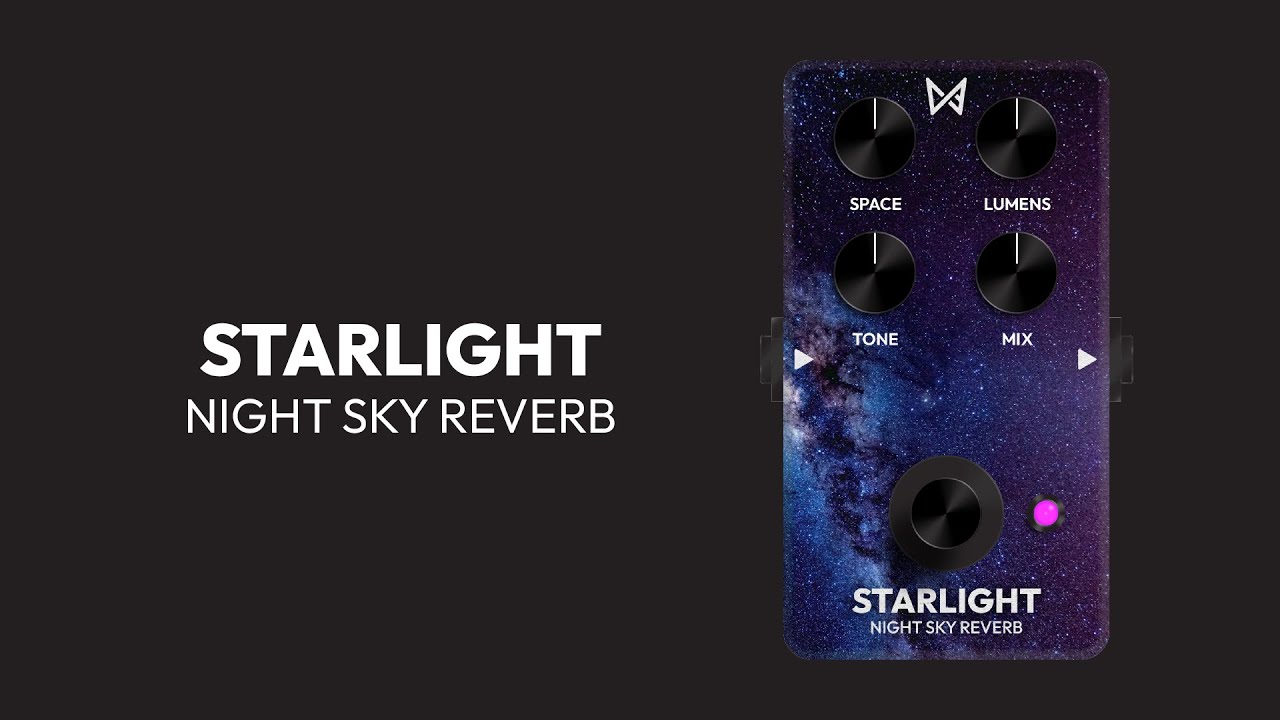The image showcases a sophisticated advertisement featuring a remote control-like device against a dark gray to black background. The left side displays the text "Starlight Night Sky Reverb" in bold white capital letters. On the right, the vertical rectangular device is designed to mimic the night sky, with a purplish-blue hue scattered with stars and a galaxy.

At the top of the device, there are four black dials arranged in a grid—two on the top row and two on the middle row. These are labeled as follows: the upper left dial is labeled "Space," the upper right is "Lumens," the lower left is "Tone," and the lower right is "Mix." Directly below these, another dial is positioned, accompanied by a fluorescent purple circle to its right, creating a striking visual element. At the very bottom of the device, the text "Starlight Night Sky Reverb" is prominently displayed in white, echoing the text on the left side of the image. The intricate design of the device, coupled with the celestial theme, suggests a high-tech piece of audio or visual equipment engineered to enhance user experience.